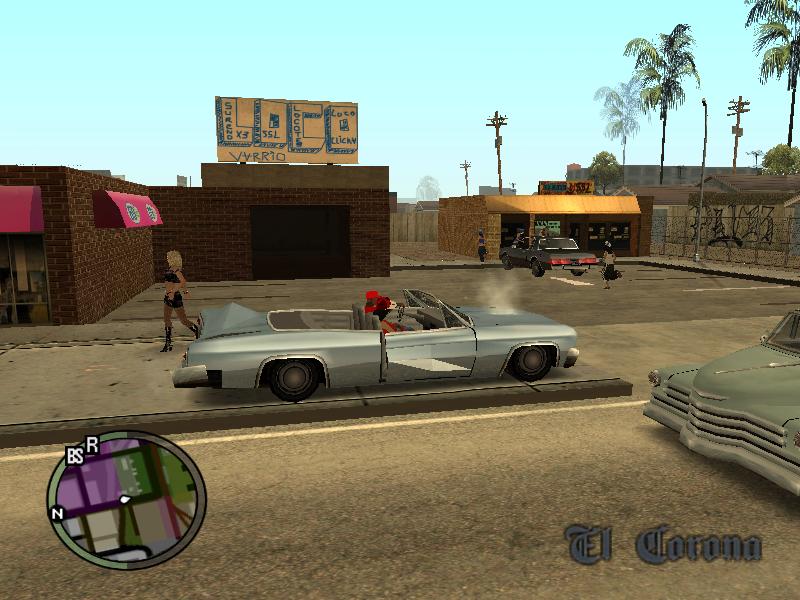The image appears to be a low-resolution screenshot from an early 2000s video game, resembling the Grand Theft Auto series. The scene depicts a gritty urban neighborhood featuring a red brick storefront with awnings—one yellow and one pink. A couple of classic lowrider cars, including a silver one with a wing and two pixelated figures in red hats, are parked along the curb. Nearby, a girl in black boots, a short skirt, and a midriff-baring top walks on the sidewalk. The backdrop includes brown buildings, one with a VVRIO billboard, and graffiti-covered walls and fences. Tall palm trees and misshapen telephone poles dot the landscape under a clear blue sky. A circular map with various symbols appears on the left side of the screen, while the gothic-style text "El Corona" is displayed in the right corner.